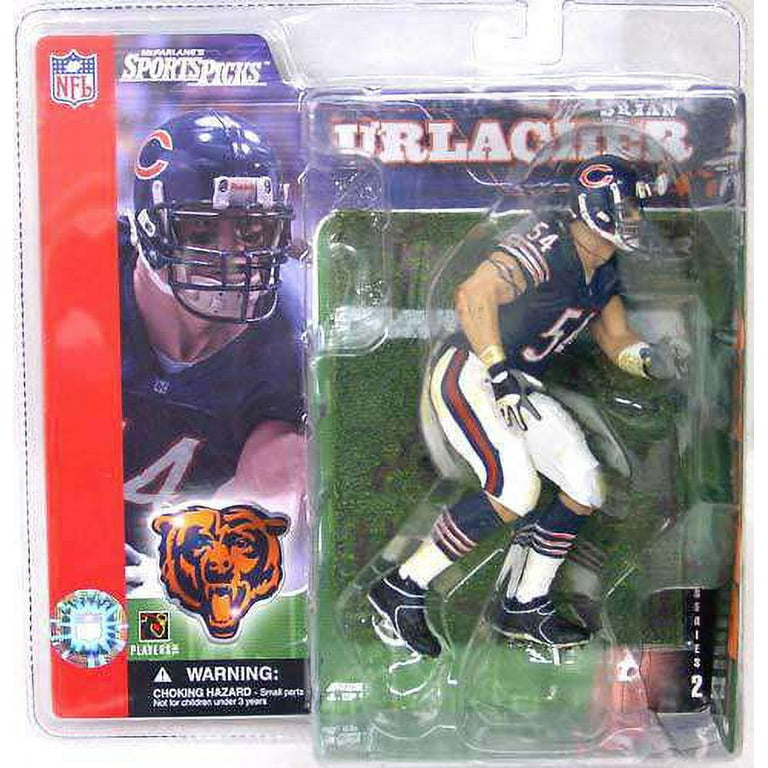This image shows a collectible action figure of renowned football player Brian Urlacher, encased in a clear plastic hanger pack designed to prevent theft and display. The figure is accurately detailed, wearing a blue helmet with a white "C" on the side and a blue jersey featuring the number 54, complemented by white shoulder stripes. He has on black, white, and gray gloves, white pants with a red stripe flanked by blue stripes, socks with blue cuffs and additional blue and white stripes, and black shoes. The packaging includes a prominent NFL logo in a red square, the McFarlane Sport Picks branding, and a warning indicating the toy is not suitable for children under three due to small parts. The backdrop showcases a green football field with white lines, while the card features a stylized image of a roaring bear—the Chicago Bears' logo. Above the figure, "Brian Urlacher" is clearly displayed, and the packaging also highlights an image of Urlacher in action, capturing his likeness and adding to the collectible's realistic appeal.